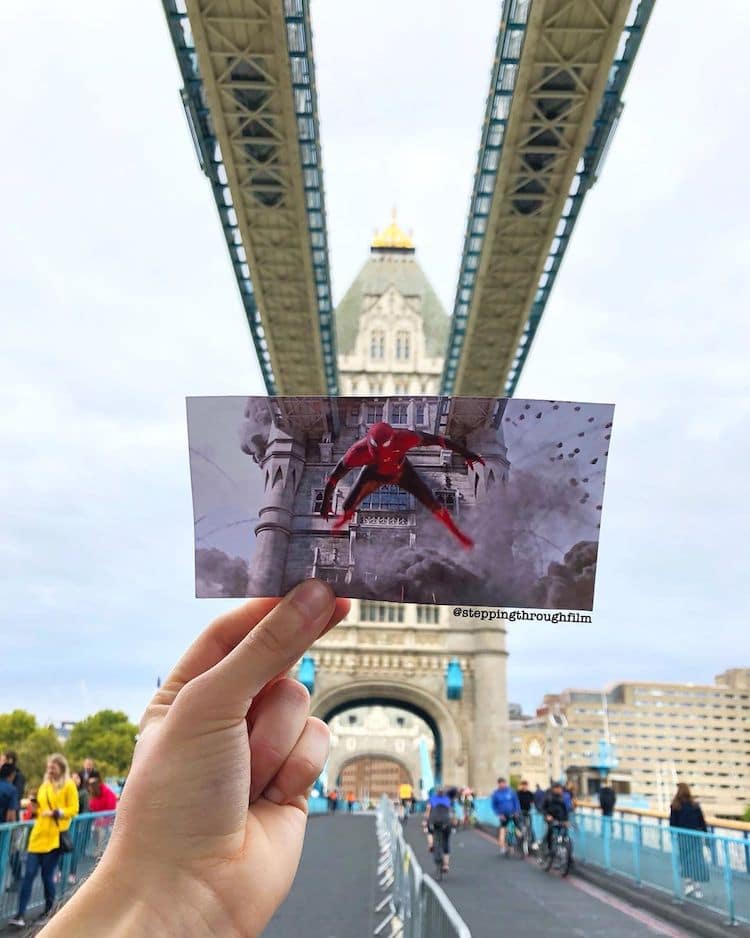In this color photograph, a person's left hand emerges from the lower left, delicately holding a photo of Spider-Man in his red leotard outfit with webbed markings and eye covers. The picture of Spider-Man, depicted mid-jump as if he were engaging with the structure, is held up precisely against a real-life scene. The background features a striking tan-colored archway that is part of a bridge, seamlessly aligned with the photo so that its dimensions match the real-life architecture. This well-known bridge has a tower with light beige stone, dual overhead walkways with blue railings, and an asphalt road lined with police barricades. Along the road, a mix of pedestrians and cyclists add life to the scene. Further in the background, other high-rise buildings of a similar tan hue, along with some trees visible to the lower left, integrate into this clever visual illusion where the fictional and real worlds blend.